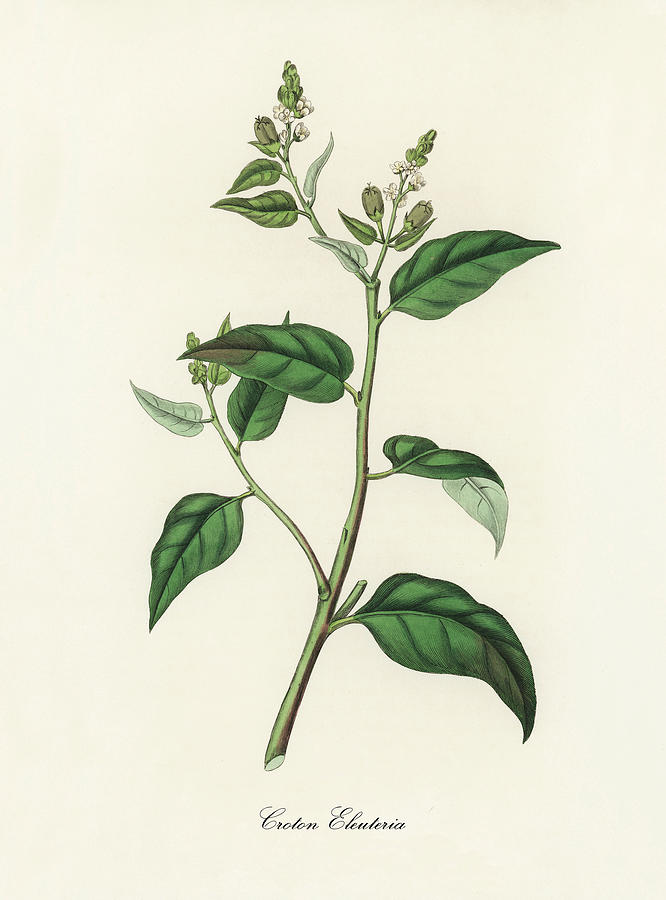This image depicts a detailed botanical illustration set against a beige background, possibly with a hint of pink. The focus is a single green plant stem that extends vertically, adorned with several side branches and foliage. At the bottom of the stem, there are two side branches, followed by additional smaller branches as one moves upward. The foliage consists of varying shades of green, from dark to light, with a noticeable large leaf at the bottom that tapers into smaller leaves towards the top. Additionally, some leaves appear to have brown edges. 

At the top of the plant, there are several buds and small flowers, which present a pinkish-white hue. A piece of text, written in cursive, is located at the bottom of the stem, potentially indicating the plant's scientific name, though it is not entirely legible. The cursive text might read something along the lines of "croton ellatoria" or "Gordon Croton Illisteria," suggesting a possible identification for the plant. The delicate and intricate details of the leaves, buds, and flowers highlight the beauty of this botanical specimen.